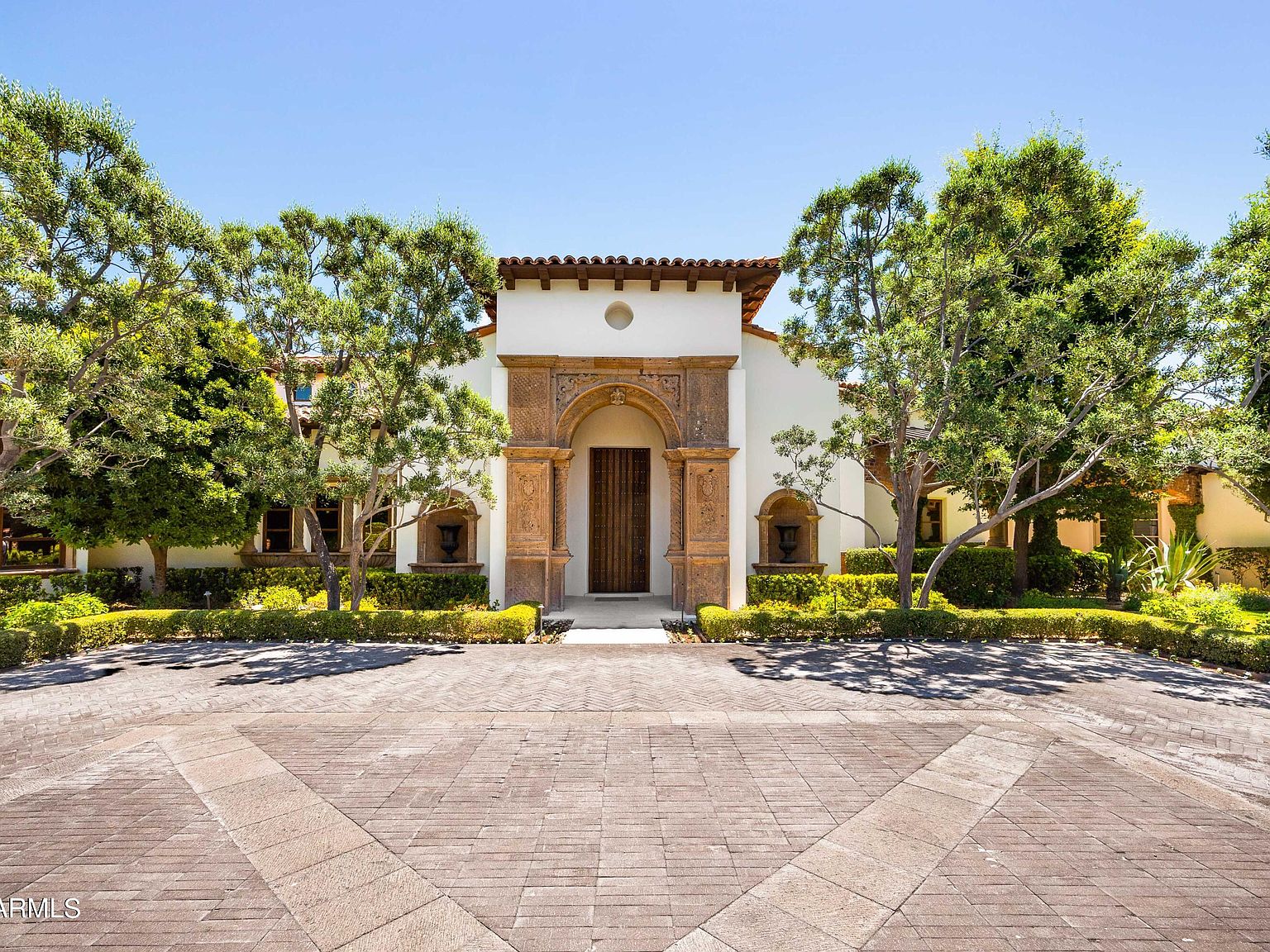This outdoor color photograph captures a Spanish-style building under a clear, bright blue sky devoid of clouds. The building, possibly a home or resort entrance, features a white or cream stucco exterior and an orange terracotta-tiled roof. The central focus is the ornate wooden door framed by a large, decorative archway with detailed molding and 3D designs. Flanking the door are symmetrical cut-out archways, each housing a statue resembling a black chalice. The building’s entrance is bordered by tall green trees and manicured shrubs, including green and yellow varieties.

In the foreground is a large, brick courtyard with reddish-gray stone tiles, extending into a wide expanse lined with hedges that border a short sidewalk leading up to a small step. This step transitions to a concrete porch in front of the archway. The courtyard is spacious and open, providing a clear view of the building's façade, which is decorated further with a circular design carved into the wall just below the roofline. 

Additionally, the bottom right-hand corner of the image bears a watermark with the text “AR MLS,” suggesting a professional photograph likely used for real estate purposes.